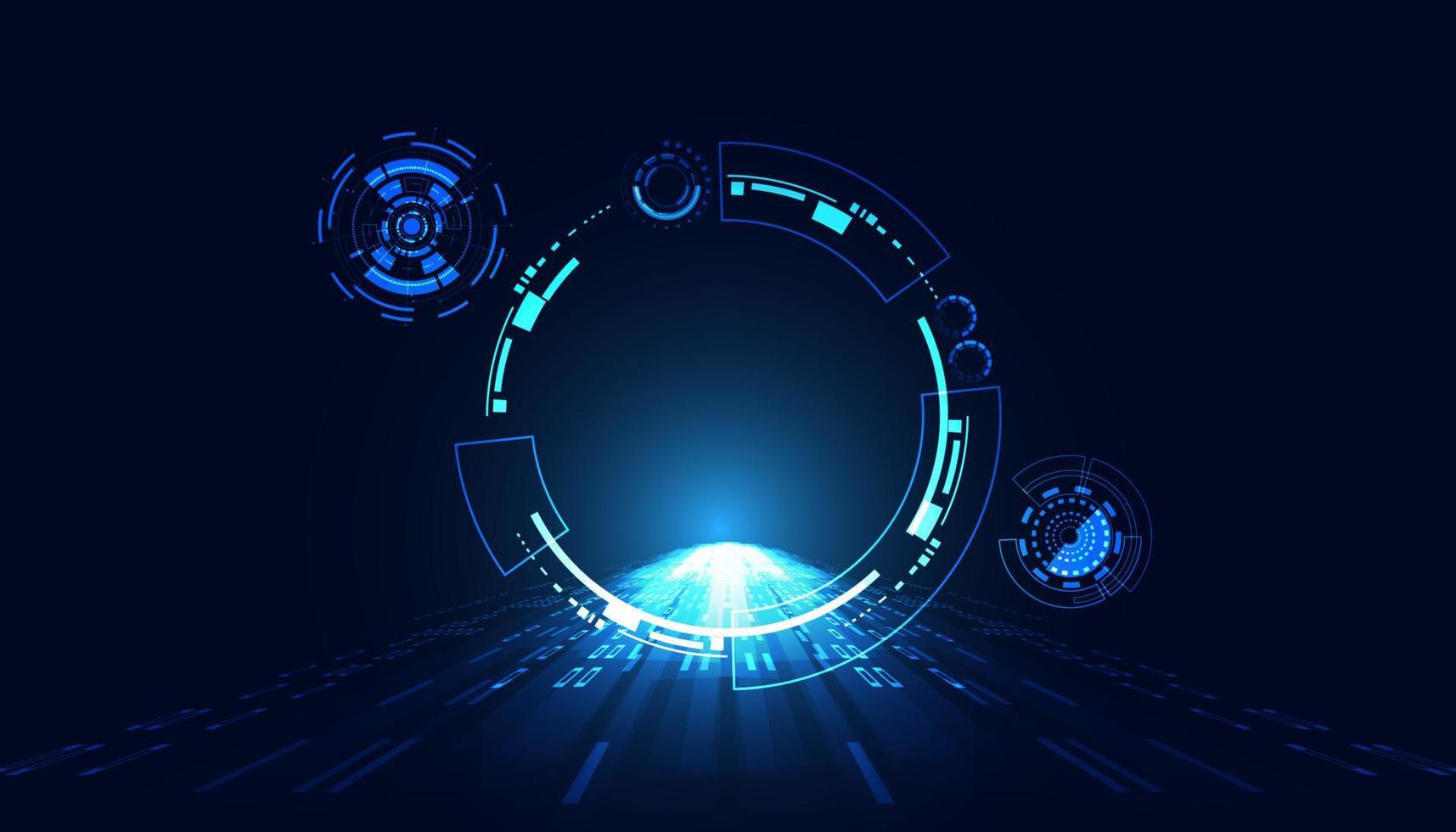This is a detailed image that appears perfect for a desktop background. The predominant theme is a dark navy blue shade, overlayed with intricate digital artwork that brings to mind a heads-up display (HUD) from a video game or a futuristic interface. The focal point is a large, central circular shape composed of dots and lines, resembling a digital readout with shades of mint green, teal, and multiple tones of blue. This central circle includes a bright, almost white flash of light in its center, suggesting a concentrated focal point or indicator.

From the bottom of the image, lines and paths of O's and other digit-like shapes — all varying in shades of light blue and dark blue — converge toward this bright center. This convergence enhances the depth and draws the observer’s eye towards the middle. Sprinkled throughout the image are smaller circles, one positioned to the upper left and another at the lower right, maintaining the same digital and abstract design motif but predominantly in blue without green elements.

The image gives off the feel of a futuristic, digital readout that might appear in a sci-fi movie or a high-tech computer game, complete with digital gauges, speed indicators, and embedded data lines. The detailed composition, combining elements of modern abstract art with digital technology aesthetics, creates an immersive, visually engaging experience.